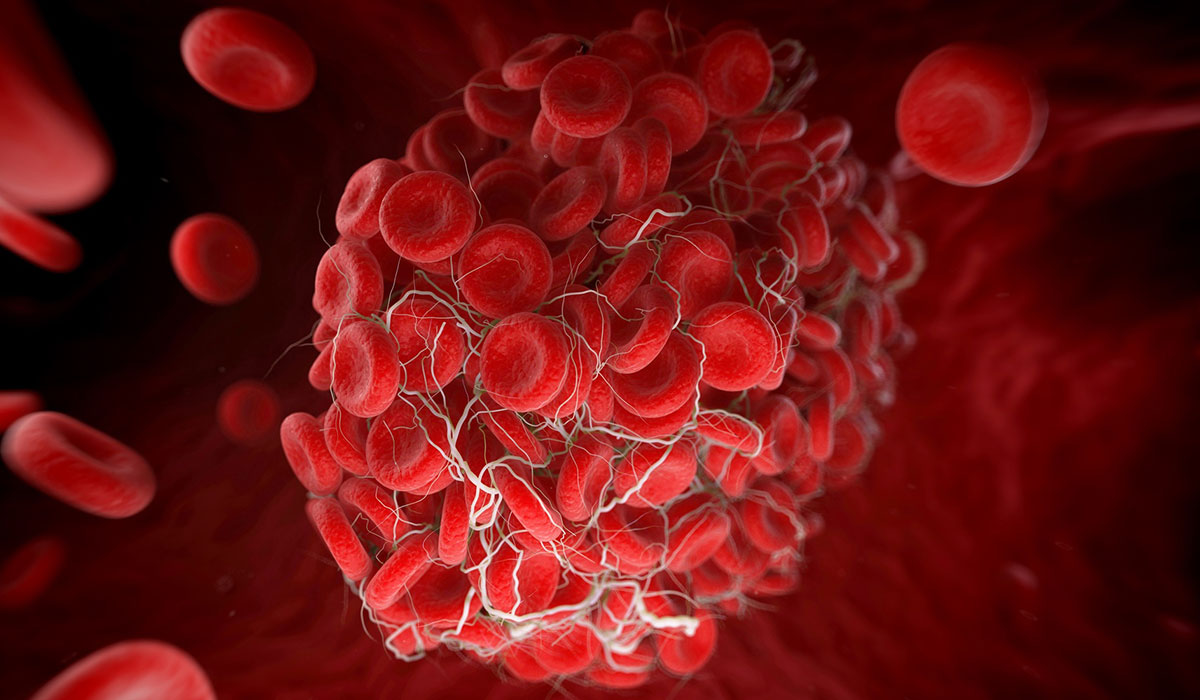This highly magnified, detailed microscopic image vividly depicts a dense aggregation of approximately a thousand red blood cells, resembling filled-in red Cheerios with distinctive central indentations. Centered within the image, these cells are interwoven with an intricate network of white stringy, web-like structures, reminiscent of shredded dental floss. Scattered around the central cluster are about ten free-floating red blood cells, with a notably large one in the upper right corner. The cells are suspended within what appears to be a richly textured, red vessel wall environment, conveying the impression of a giant red sponge in the background, along with some indistinct darker areas. The overall scene, resembling both a scientific photograph and an artistic close-up, combines the rough texture of the cell surfaces with a visually striking contrast between the clustered and individual cells against the blurred, red backdrop.